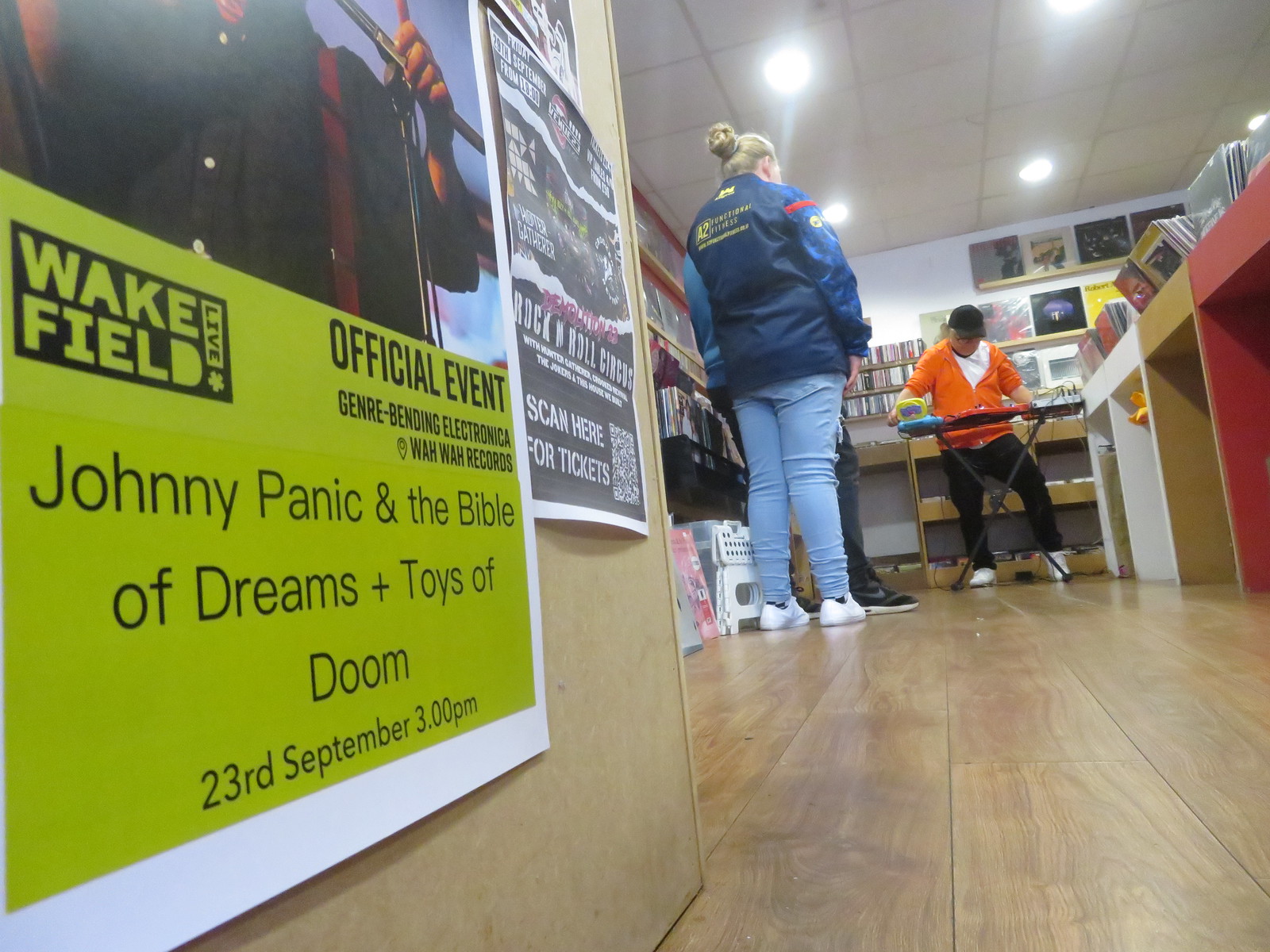In this photograph taken from near the ground, the scene captures the interior of what appears to be a music store. The setting features 3-4 people, gathered around a central figure who is enthusiastically playing a keyboard. The floor is a rich, light brown hardwood, while the ceiling is adorned with square tiles illuminated by four bright white lights.

The left wall is decorated with various posters, including a prominently displayed sign reading, "Wakefield Live - Johnny Panic and the Bible of Dreams plus Toys of Doom, 23rd September, 3pm, Official Event, John Ray Bending Electricana." This wall adds a touch of vibrant color with shades of tan, green, black, red, orange, purple, dark blue, yellow, and light blue reflecting the diverse merchandise.

On the right side of the room, rows of shelves are filled with items that appear to be album records or perhaps other collectibles, contributing to the nostalgic ambiance of the store. In the center, a woman with her blonde hair styled in a bun, dressed in a blue jacket and light blue pants, stands with her back to us, partially obstructing another individual whose leg is just visible.

Another person stands to the right, facing the camera from behind a table, donning a black cap, an orange sweater over a white t-shirt, and black pants. Behind him, the wall features more hanging items, likely records, enhancing the musical theme of the store. Adjacent to this setup is a table in the foreground, showcasing an array of records or books displayed upright, adding a structured yet casual element to the scene. The room's wooden floor frames the entire image, grounding the eclectic yet harmonious arrangement of people and objects within this vibrant indoor setting.